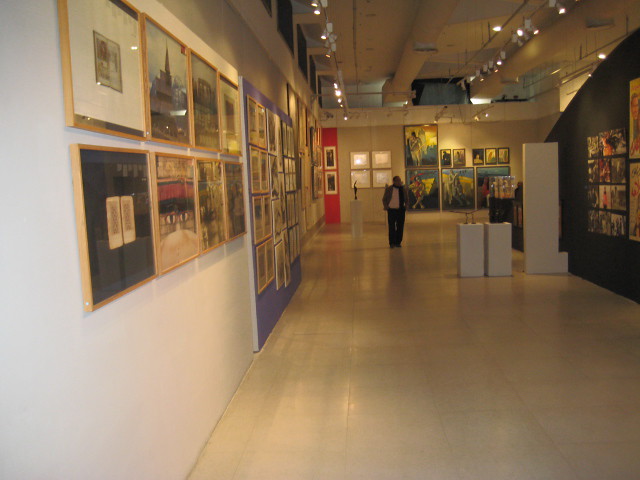The photograph captures the interior of an art gallery or museum with a tall, roughly 20-foot ceiling featuring exposed cylindrical pipes and rail-mounted fluorescent lighting. The space is characterized by a white-tiled floor and predominantly white walls adorned with various framed artworks. On the left wall, several pictures are arranged in a linear fashion, while the far wall features a red section amidst more artwork. The right wall and a corresponding black staircase, which curves downward, also display framed pieces. Near the center of the room stand white pedestals supporting exhibition pieces that are indistinguishable due to their distance. A solitary figure can be seen walking along the hallway, further enhancing the scale and depth of the space. The scene is illuminated by strategically positioned lights pointing at the walls, enhancing the visibility and ambiance of the exhibited works.